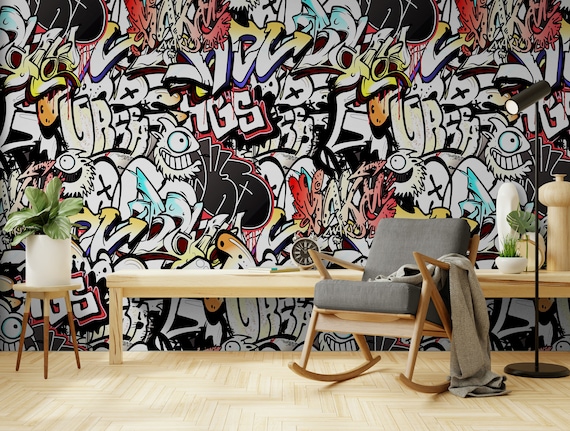This image depicts a unique living room featuring vibrant graffiti art on the main wall. The wall is adorned with professionally done, colorful graffiti that includes various images, cartoonish creatures—such as one-eyed monsters and stinging fish—as well as numerous tags and letters. The dominant colors in the mural are red, white, blue, and yellow. 

The room is furnished with all-wood pieces contributing to a modern yet cozy ambiance. On the left side, there is a wooden stand holding a white vase with a small green house plant. Adjacent to it is a long, low wooden bench. A wooden rocking chair with a gray cushion and a tan blanket draped over its left armrest sits beside a black lamp on a slender pedestal. Another table holds additional potted plants and decorative wooden items. The floor features a clean, herringbone pattern in tannish wood, adding to the room's warm atmosphere. Overall, this appears to be an eclectic yet inviting space where art and home comfort beautifully merge.